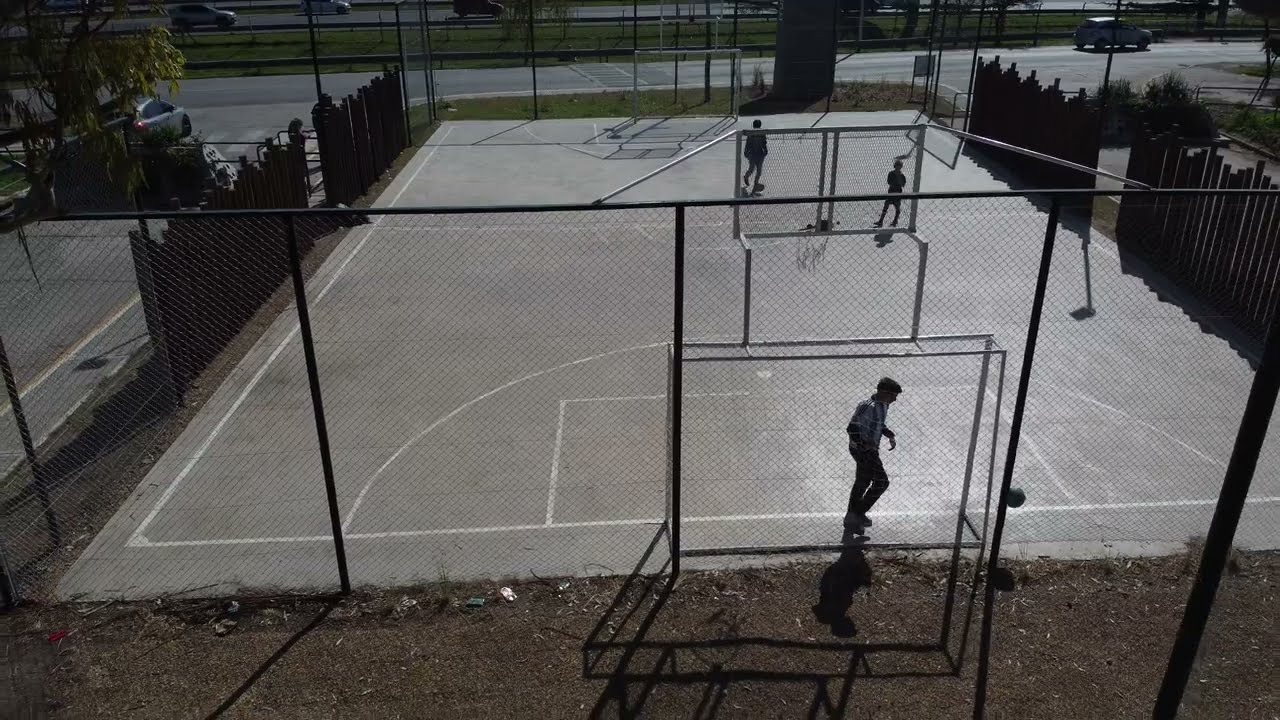This image captures an outdoor basketball court, which is paved with gray cement and marked with white lines. The court is surrounded by a substantial fence, possibly wooden, providing a enclosed playing area. Two basketball hoops stand at either end of the court. The scene includes three people; one man is standing under a hoop, heading towards a bouncing basketball, while the other two figures are positioned towards the back of the court, suggesting they may be engaged in some activity. The area appears somewhat shadowy and not particularly clear, suggesting an overcast or dusk setting. Beyond the court, a roadway is visible with a moving vehicle and parked cars, hinting at nearby parking facilities. The surrounding environment looks somewhat neglected, with litter scattered around. The court is set amidst dead grass, adding to the somber tone of the scene.